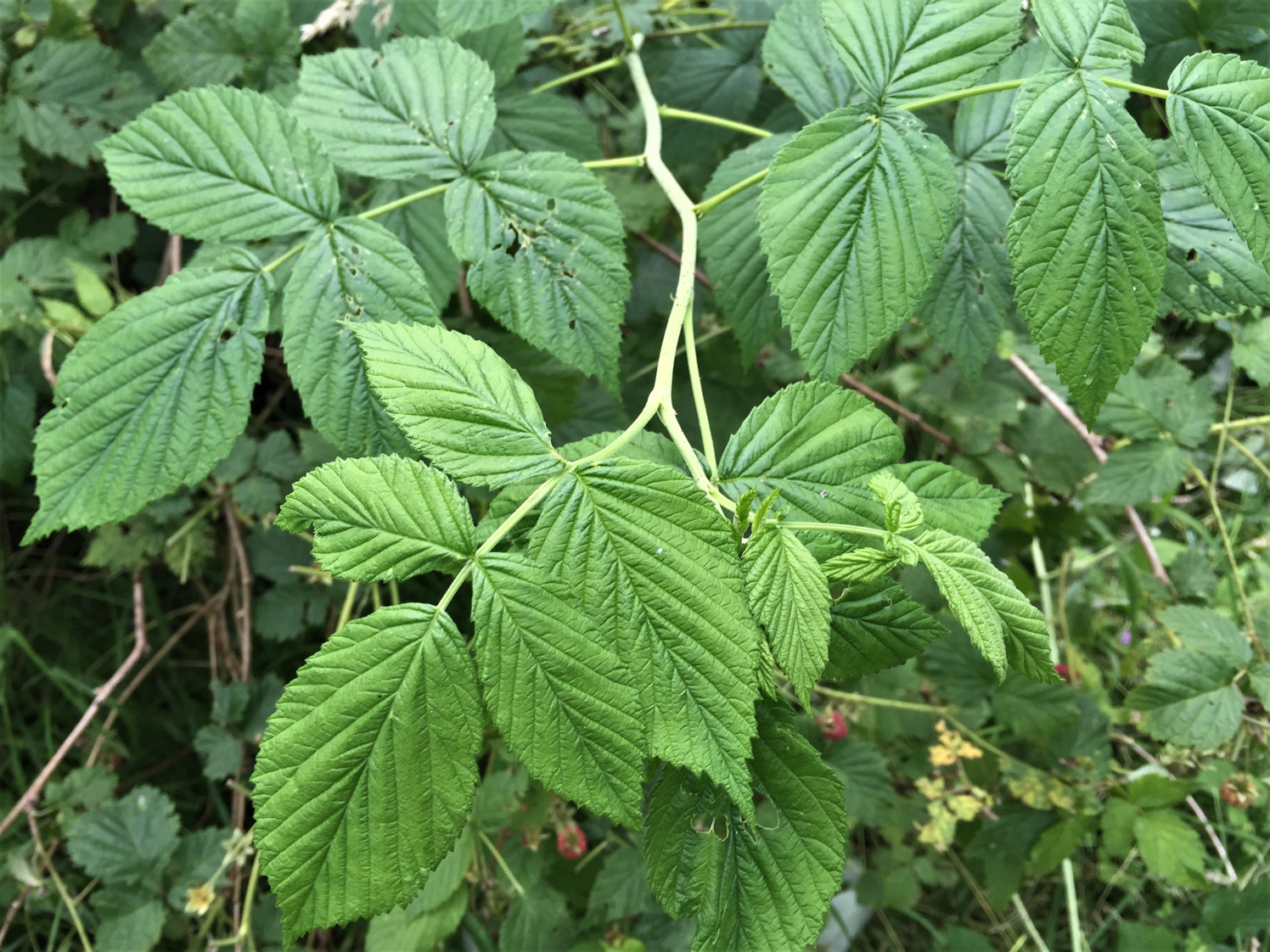This close-up photograph captures a verdant scene dominated by a lush, wild raspberry bush. The focus is on the dense, overlapping green leaves, which are mostly oval-shaped and slightly pointed. Amidst this greenery, small red raspberries and tiny flowers can be seen, hinting at a thriving plant in different stages of growth. Stems are visible branching through the leaves, some appearing whitish while others are green. A closer inspection reveals some leaves displaying signs of decay, turning yellowish-brown or having small holes. The photograph, taken on what appears to be a cloudy day, lacks strong sunlight, giving the scene a softer, more diffused light. While it is difficult to ascertain the exact location, the wild, untamed nature of the bush suggests it could be found in a wooded area or possibly a neglected garden. The overall impression is one of natural, chaotic beauty, with leaves and branches sprawling in all directions.